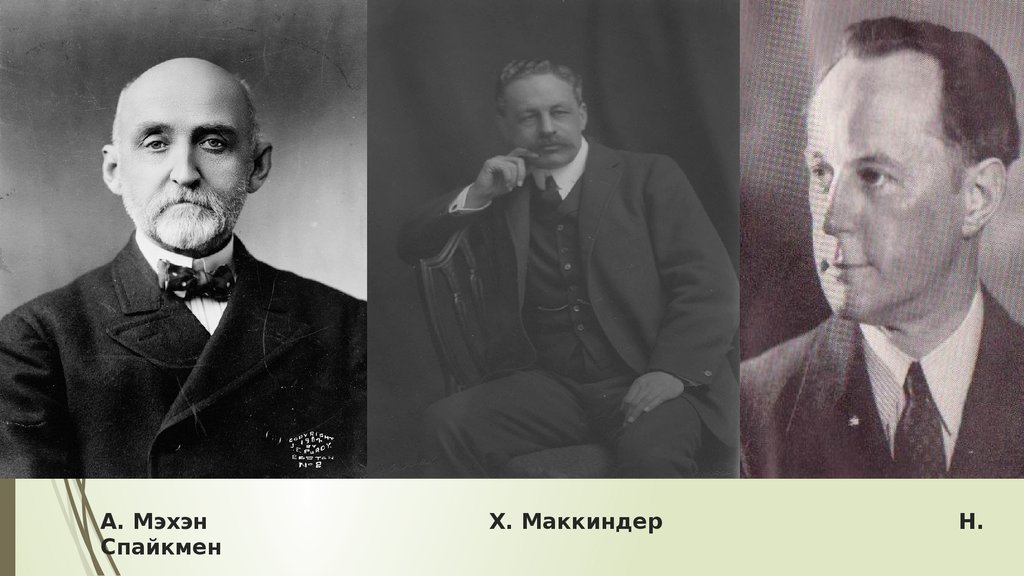The black-and-white image displays three older men, their portraits lined up side by side. Each man is dressed in a suit, illustrating a historical and formal ambiance. The first portrait shows a bald man with a beard, adorning a dark suit and bow tie. The text below him appears to be in a foreign or possibly stylized format, closely resembling "A. Mexicanecami." The middle portrait is of a man with a mustache, seated in a chair in a contemplative pose, one hand on his chin and the other resting on his lap. The text underneath this image reads "X. Macaca." The third portrait features a clean-shaven man gazing to the left, wearing a dark suit with a white shirt and tie, captioned with the initial "H." The coherence in their attire and the monochromatic tones suggest this might be a politically or historically significant image.